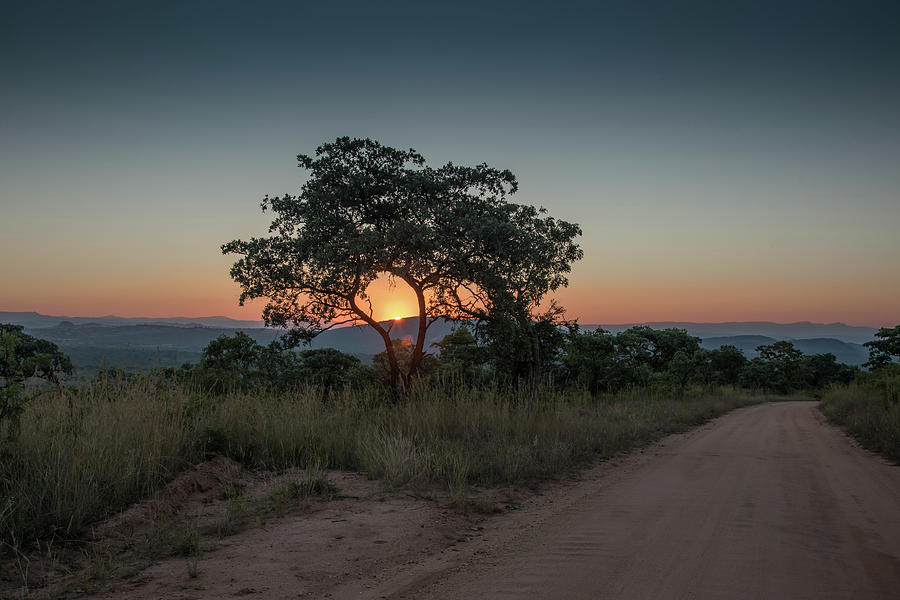The image captures a serene nature landscape during either sunrise or sunset, with the sun appearing majestically through the branches of a large central tree. This tree stands prominently in the middle of the frame, showcasing two distinctive branches extending left and right. The sun bathes the scene in a warm, glowing light of orange and yellow hues, blending into a darker blue and grey sky. Towards the horizon, an expanse of blue mountains stretches across the background.

On the right side of the image, a muddy dirt road weaves its way through the scene, curving into the middle distance and flanked by green grass and brush. The road, tan in color due to the sand, is devoid of vehicles, enhancing the tranquility of the setting. Surrounding the central tree are several other dark green leafy trees, adding depth to the verdant landscape. The earth-toned vegetation and maintained pathways suggest a well-preserved natural area, inviting viewers to appreciate the outdoor beauty.